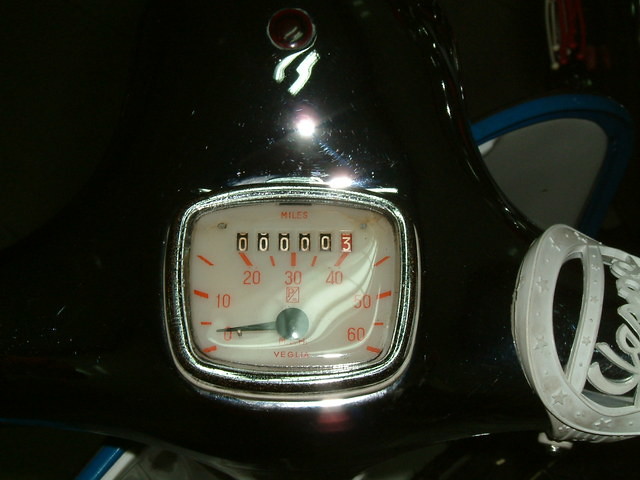A detailed close-up photograph of a vintage speedometer, likely from a Vespa scooter, takes center stage. The rectangular speedometer with rounded corners is framed by a chrome bezel, positioned slightly below center and to the left of the image. The dial of the speedometer spans from 0 to 60, highlighting every multiple of ten (10, 20, 30, 40, 50, 60) with dashes in between. The needle points to zero, against a black backdrop.

Directly below the speedometer, the odometer reading is visible, showing "00003" miles in five-digit format. Above the odometer, the word "miles" is printed in orange. The right side of the frame hints at a silver crest, partially obscured but possibly reading "Vespa." The backdrop of the image is predominantly black, with two noticeable flash glares positioned above the speedometer. To the right of the chrome bezel, a faded blue and white element can be partially seen in the background. No additional text or markings are visible in the photograph, focusing attention on the classic design and details of the speedometer.